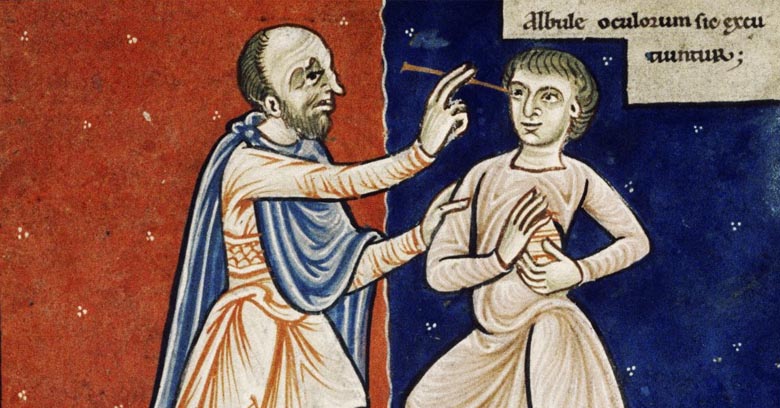This image is a detailed medieval painting in the style of an illuminated manuscript. The scene is divided into two distinct background panels. A red panel with yellow dots serves as the backdrop for the left side, while a blue panel with white dots is on the right. In the foreground, we observe two male figures. 

The man on the left, positioned in profile looking right, is clad in an orange robe secured by a clasp, over which he wears a blue cloak. This figure is bald, has white skin, and is depicted with a notably long nose. He is holding what appears to be a stick or needle, pointing it towards the eye of the other figure. His overall appearance is aged and his attire suggests a representation of wisdom or authority.

Facing him on the right is a younger man with long, black hair. Dressed in a brown robe, he clutches an object in his hands and seems to be warily receiving the intervention of the man on the left. This figure is set against the blue background panel.

Above the scene is a line of Gothic text, "ALBULEOCULORUMFICEXCUWAUNTUR," which appears to be an archaic script, possibly a Biblical reference, hinting the parable about the mote and the beam in one’s eye. The script is in Gothic print, giving a strong medieval manuscript feel to the image.